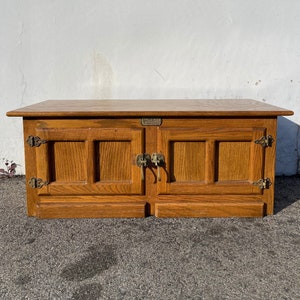The image features an outdoor scene showing a piece of wooden furniture placed on a gray cement pavement next to a light cream or white wall. This furniture, resembling a TV stand or shelving unit, is crafted from a shiny, golden brown finished wood. The structure is rectangular, with a flat top that slightly extends over the base. Below the top, there are two large cabinet doors, each framed by recessed wooden panels with a central dividing line, adorned with brass door handles. Metal latches and silver hinges on the sides allow these doors to open, offering storage space within. The pavement beneath, where the furniture sits, displays a darker, wet-looking spot, possibly oil stains. The scene evokes a sense of an item temporarily removed from an interior setting, perhaps placed next to a shed or garage.